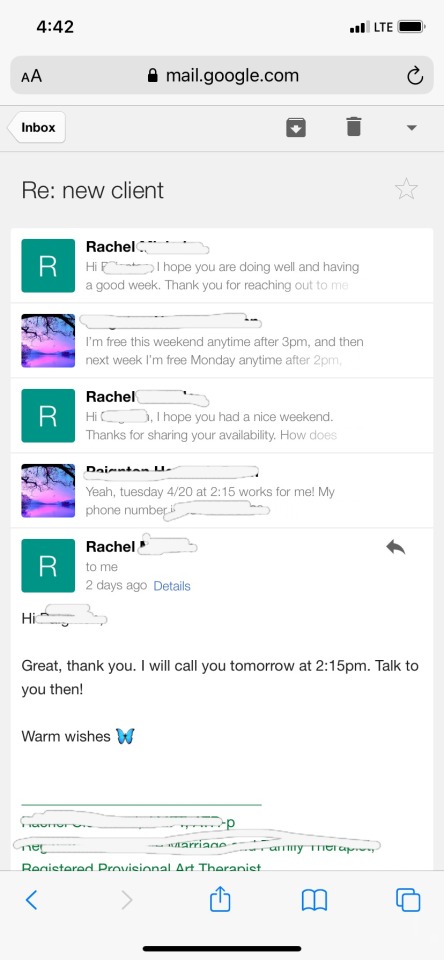This image captures a screenshot from a cell phone, showcasing an email conversation on a grey and white background with black text. In the upper left corner, the time reads 4:42. On the upper right, icons for Wi-Fi and battery status are visible. The top of the screen displays a lock symbol, indicating a secure site, followed by the URL mail.google.com and the label "Inbox" in the upper left.

Directly under this, within a grey area, the text "RE: New Client" appears in black. Below, in a white messaging area, are email exchanges featuring different participants. A green square with a white "R" indicates messages from Rachel, whose last name is crossed out. Her message reads, "Hi [name crossed out], I hope you're doing well and having a good week. Thank you for reaching out to me."

The reply is from someone with a profile picture showing a purple sunset with a tree. Their name is also crossed out. The message reads, "I'm free this weekend, anytime after 3 p.m. Next week, I'm free Monday, anytime after 2 p.m." Rachel then replies, "Hi [name crossed out], I hope you had a nice weekend. Thanks for sharing your availability. How does..." followed by more text.

The conversation continues with the other person confirming, "Yeah, Tuesday, 4/20 at 2:15 works for me. My phone number is [number crossed out]." Rachel responds, "To me," and another part reads, "Hi [name crossed out]." The talk concludes with, "Great, thank you. I will call you tomorrow at 2:15 p.m. Talk to you then. Warm wishes," followed by a butterfly emoji. Several elements at the bottom of the screen are crossed out for privacy.